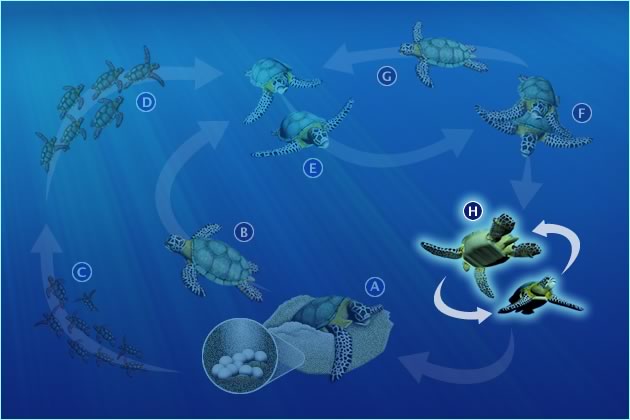This infographic depicts the life cycle of sea turtles through a sequence of stages, with alphabetical labels A to H, set against an underwater backdrop illuminated by sun rays from the upper left. The diagram begins at stage A, showing a turtle laying eggs in a nest among rocks. Stage B captures the moment when both the mother turtle and the newly hatched baby turtles swim away. At stage C, the baby turtles join a larger group, indicating their early life in the ocean. Moving to stage D, the turtles are shown growing larger, continuing their journey through the waters. In stage E, the turtles have reached a decent size, highlighting their maturation. Stage F illustrates the mating process, with one turtle positioned on top of another. This is followed by stage G, where one of the turtles swims off alone. Finally, stage H depicts two adult turtles swimming together, completing the cycle. The overall diagram visually narrates the journey from eggs to adulthood within the aquatic environment, capturing both individual and communal aspects of a sea turtle's life span.